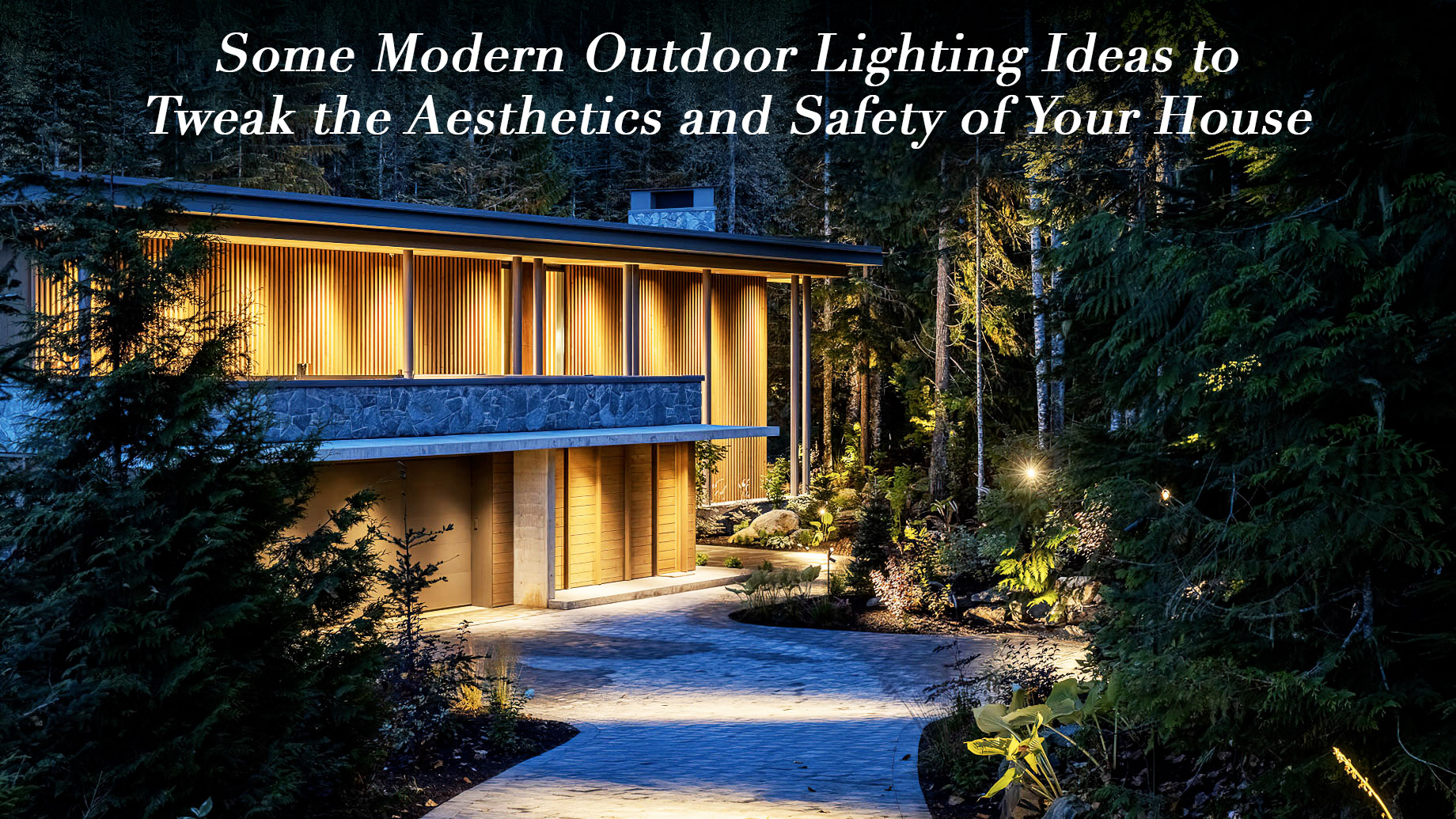The photograph captures a detailed outdoor scene featuring a two-story building prominently on the left side. The building, constructed with light brown walls, includes a flat roof and a gray balcony on the first floor, supported by pillars. To the right, a mixture of empty ground area and lush greenery with numerous plants and trees encircles the structure, creating a natural frame. Among the verdant foliage, dark green evergreen trees are distinctly visible. A sidewalk is positioned at the bottom center, meandering towards the building before redirecting towards the adjacent forested area on the right, rich with various trees. Illuminating the scene, several bright yellow lights suggest it’s approaching dusk. At the top of the image, a serif italicized text in white letters reads, "Some modern outdoor lighting ideas to tweak the aesthetics and safety of your house."